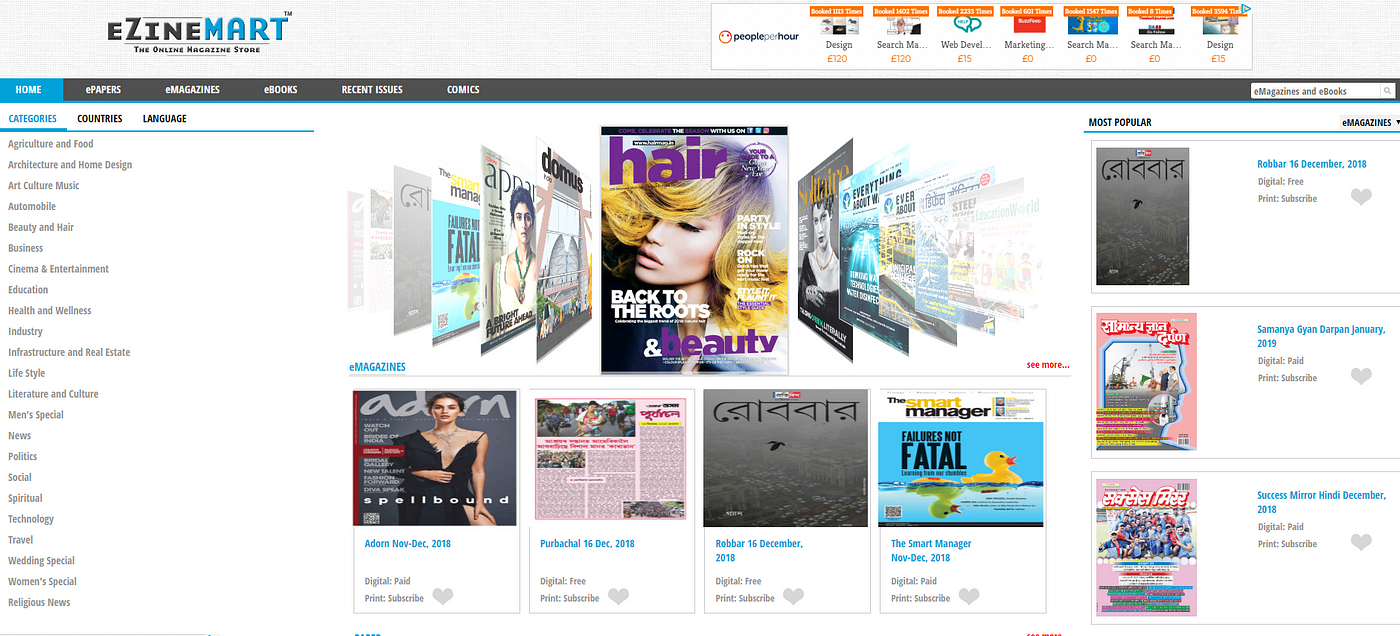The image features a webpage for "E-Zine Mart," an online magazine store. The top of the page prominently displays the store's name and tagline, "The Online Magazine Store." The website offers a comprehensive navigation menu, including categories such as Home, E-Papers, E-Magazines, E-Books, Recent Issues, and Comics. 

Under the main categories, there is an extensive list of genre-specific options including Agriculture and Food, Architecture and Home Design, Art, Culture and Music, Automobile, Beauty and Hair, Music, Cinema and Entertainment, Education, Health and Wellness, Industry, Infrastructure and Real Estate, Lifestyle, Literature and Culture, Men's Special, News, Politics, Social, Spiritual, Technology, Travel, Wedding Special, Women's Special, and Religious News.

The central section of the page showcases various magazine covers. A highlighted cover is "Hair Magazine," featuring a model with blonde, wavy hair, accompanied by the text "Back to the Roots" and "Beauty" in purple letters. Other notable magazine covers displayed include "Adorn Magazine," and "The Smart Manager." The latter features an image of rubber ducks and the headline "Failure is Not Fatal."

Overall, the layout and design suggest a user-friendly online shop, offering a diverse range of magazines for purchase across numerous interests and categories.